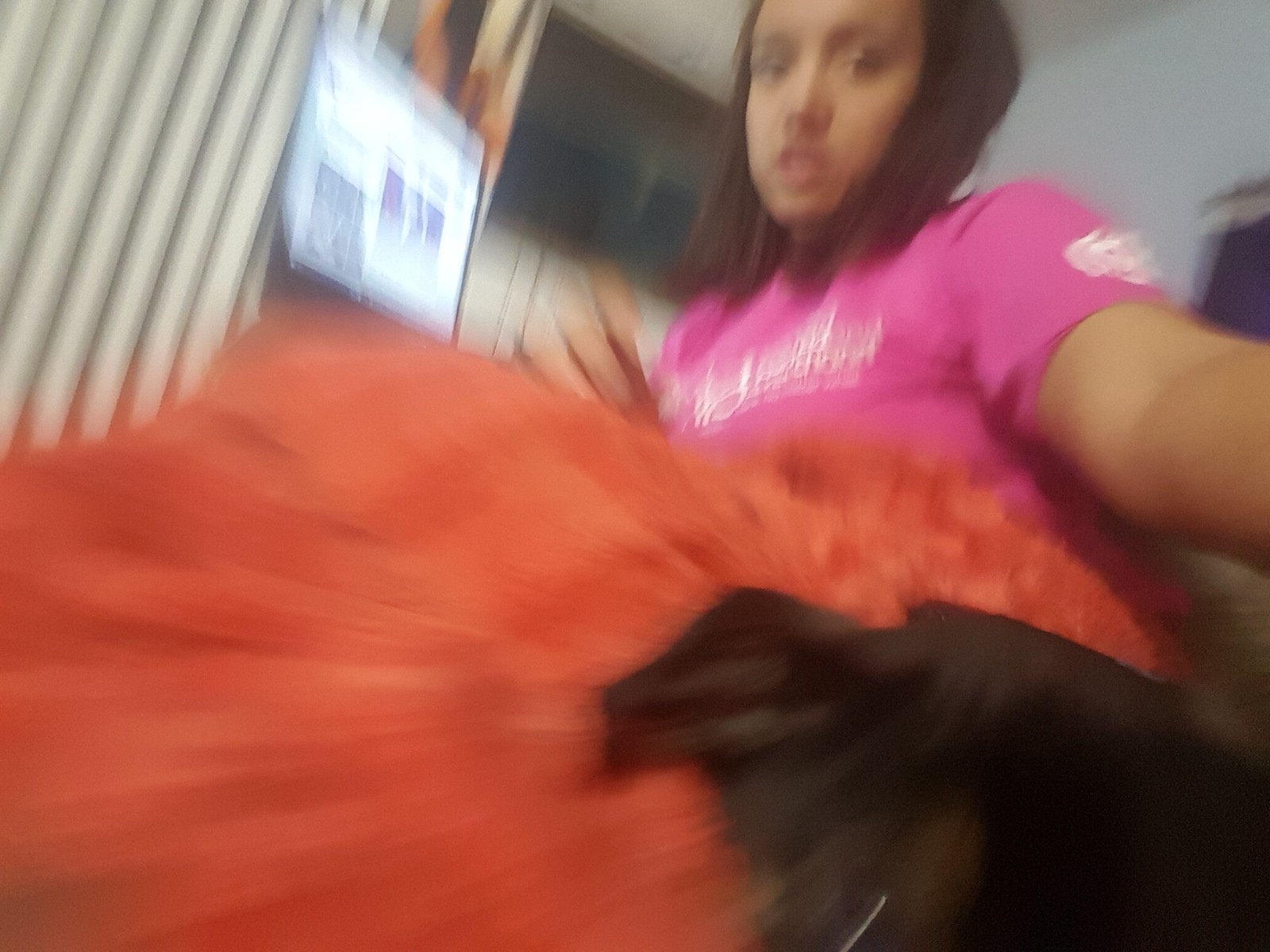This photograph captures a young teenage girl taking a selfie. She is dressed in a bright pink t-shirt adorned with white lettering across the chest. Her dark brown hair falls to her shoulders. Despite the significant blur - likely caused by her movement while capturing the image - her intent gaze towards the camera remains discernible. The girl seems to be holding the camera at arm's length, aiming it directly at her face. She appears to be wearing a bright orange skirt featuring ruffles, though it might alternatively be a colorful blanket draped over her. In the dimly visible background, a glowing screen - possibly a tablet, computer, or TV - suggests a social media feed or application. To the left, vertical blinds cover a window, and the walls behind her are painted a simple white, adding a soft contrast to the vibrant hues of her attire.